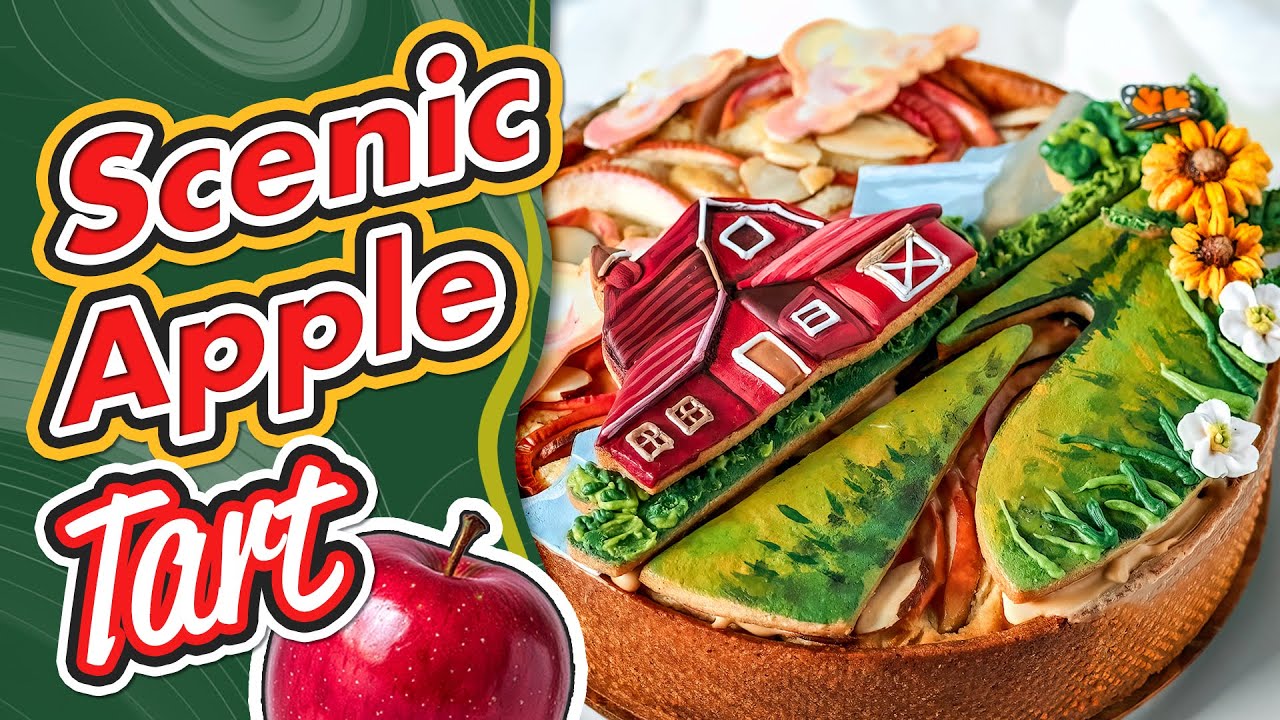The image features a stylized, graphic design advertisement for a "Scenic Apple Tart." On the left side, within a squiggly green background, the red cursive text reads "Scenic Apple Tart," accompanied by an illustration of a red apple highlighted in white. The right side of the image showcases the tart itself, set on a white surface. The tart is intricately decorated with a 3D-like frosting depicting a picturesque red barn with white outlines, sitting on lush green grass. In front of the barn is a small, empty field, and vibrant sunflowers dot the landscape. Sliced apples are interspersed with various types of crackers, completing the elaborate design. Above the barn, fluffy clouds enhance the idyllic scene.